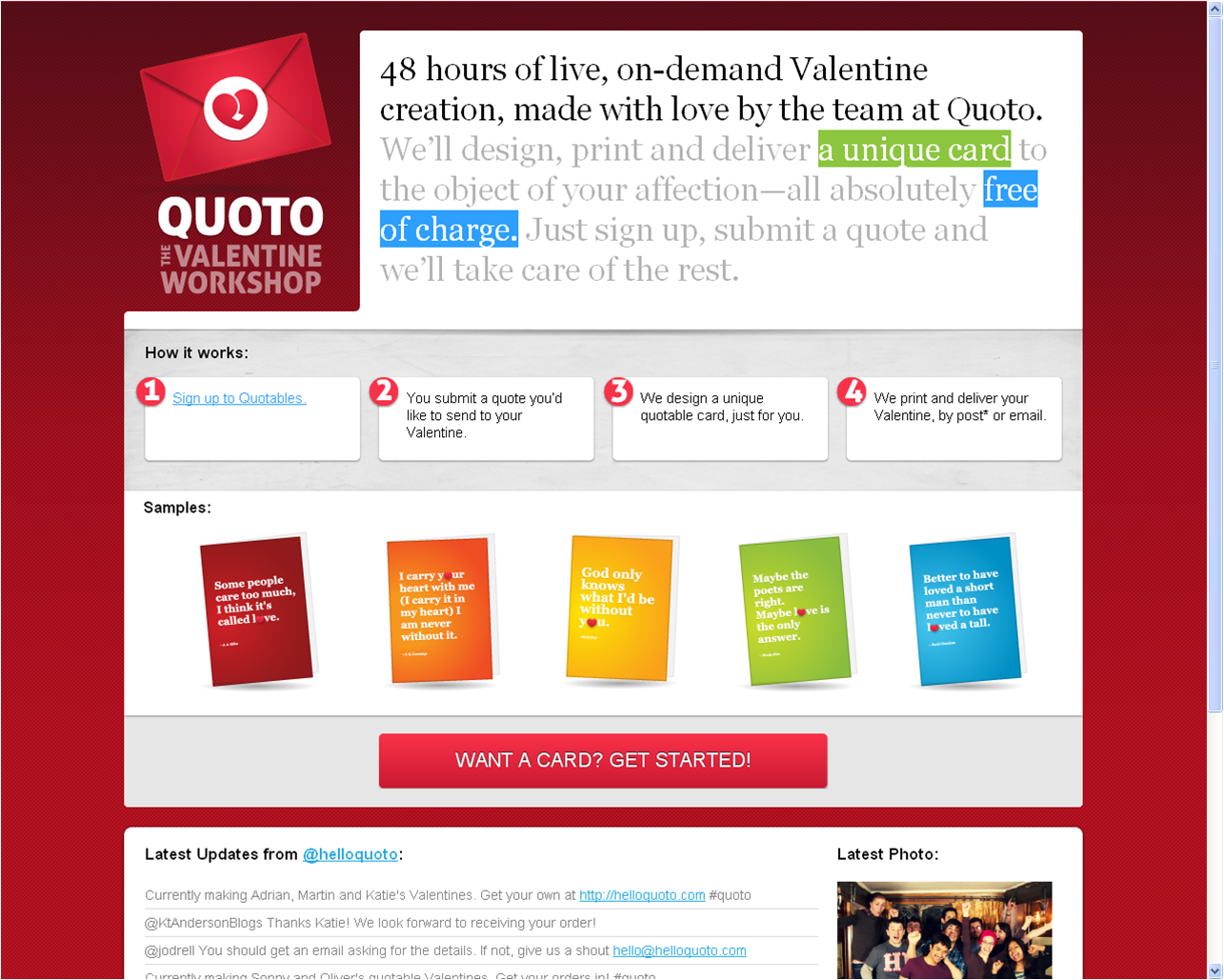The image is a screenshot of a webpage from "Quoto: The Valentine Workshop." The prominent feature of the page is Quoto's emblem, a red envelope with a heart, right next to a text box. The background of the page is a solid red color, contrasting with white text elements.

At the top of the page, a headline reads: "48 hours of live on-demand Valentine creations made with love by the team at Quoto." Below the headline, a detailed description explains the service: "We'll design, print, and deliver a unique card to the object of your affection. All absolutely free of charge. Just sign up, submit a quote, and we'll take care of the rest."

The process is outlined step-by-step in a horizontal sequence of four boxes:
1. Sign up to Quoto.
2. Submit a quote you'd like to send to your Valentine.
3. We design a unique quotable card just for you.
4. We print and deliver your Valentine by post or email.

Additionally, the page features samples of five colorful cards. The sample cards are colored red, orange, yellow, lime, and blue. The red card contains a quote that starts, "Some people care too much. I think it's called love." While the other quotes are partially visible, they are too small to read clearly.

At the bottom of the page, there's a call-to-action box stating, "Want a card? Get started!"

Overall, the webpage is an engaging and vibrant promotion of Quoto's free Valentine card creation service, featuring easy-to-follow steps and colorful card samples.